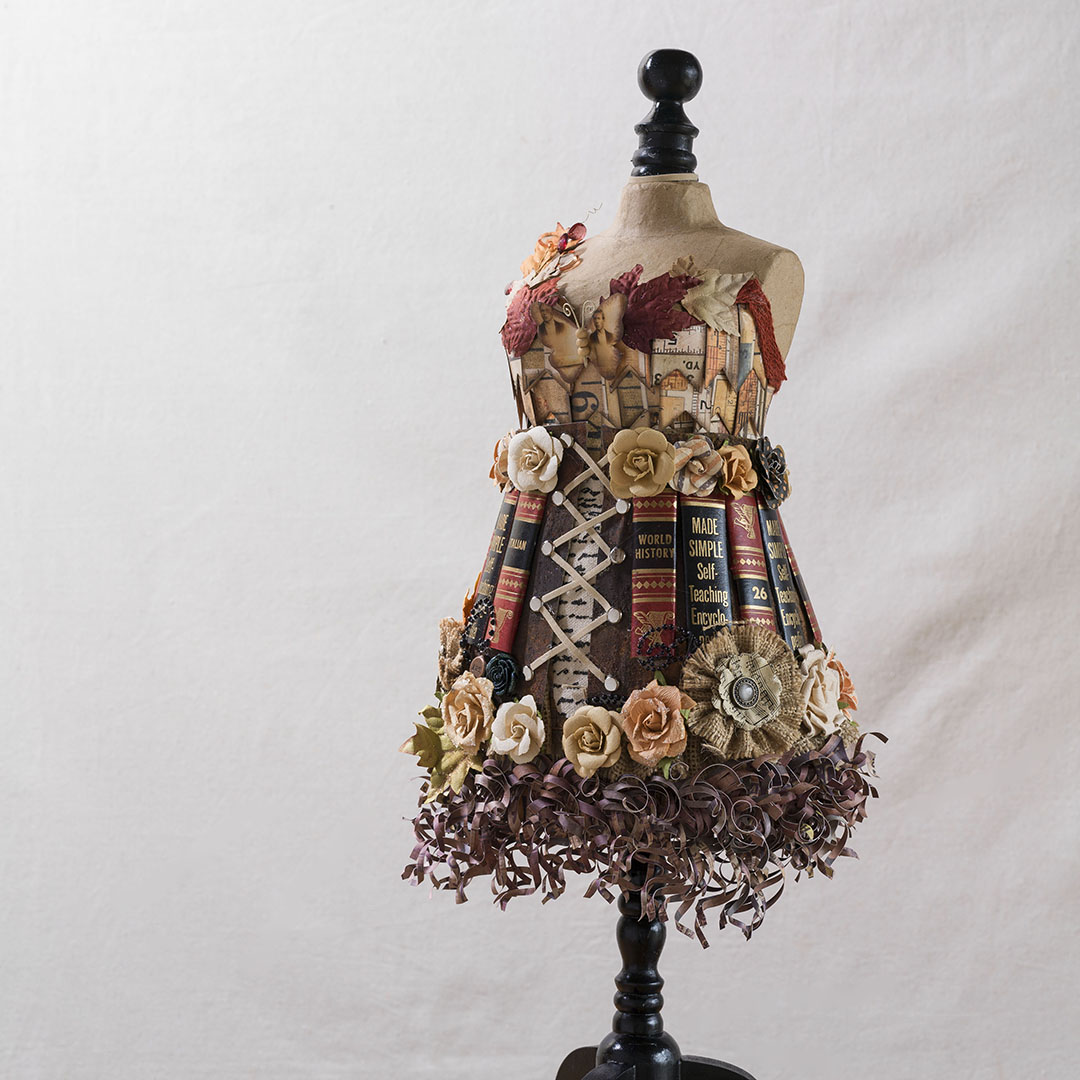This photograph captures a uniquely ornate dress displayed on a black wooden pedestal, which features a mannequin top that ends just below the neck and shoulders. The sleeveless dress, which falls to about knee-length, stands out due to its intricate construction primarily using bookbindings. These bindings, adorned with various texts like "World History Made Simple" and "Self-Teaching," bring a vibrant mix of red, blue, brown, black, and yellow hues accented with gold lettering, contributing to the dress's multicolored appearance. The skirt section is characterized by pleated designs, with each pleat presenting a different pattern.

The middle of the dress is adorned with large silk or ribbon flowers, as well as additional flowers around the waist, which also features a noticeable buckle. The bottom hem of the dress sports curled paper or wood shavings, evoking the appearance of coiled ribbons interspersed with roses or other silk flowers. A criss-cross string pattern reminiscent of a corset runs down the center, adding an intricate detail to the design. The entire ensemble is photographed against a white background, suggesting a professional setting that highlights the dress's fascinating and eclectic artistry.